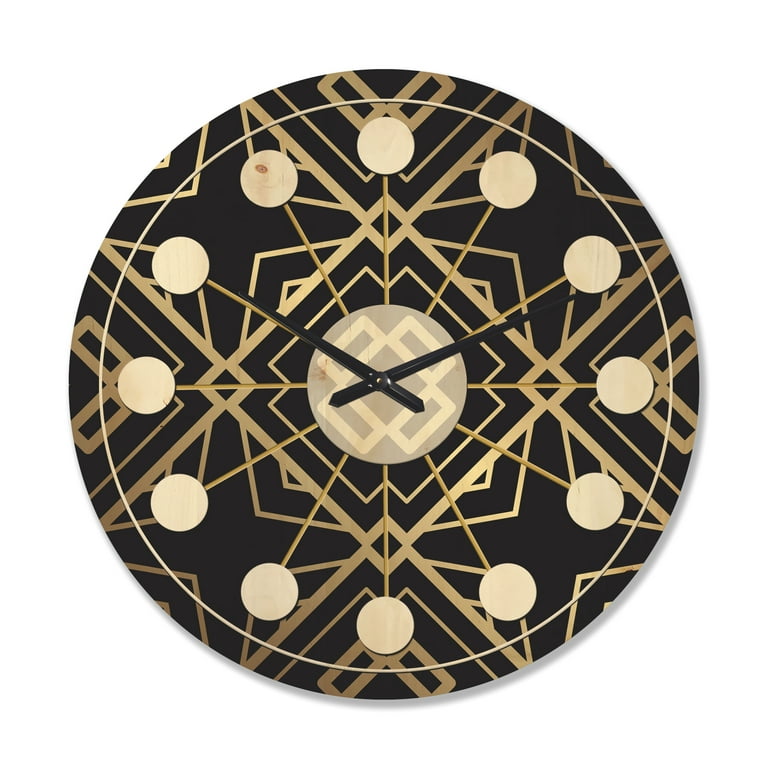This striking and modernistic wall clock features a bold Art Deco design with a round face devoid of traditional numbers. Instead, the hours are marked by small tan or light-colored wooden discs mounted on dowels, adding a unique three-dimensional effect. The clock's background is a deep, rich black, intricately adorned with a variety of geometric shapes in a shimmering gold tone, including rectangles, squares, triangles, and star-like patterns. These shapes are arranged in a repeating pattern, with a central square graphic from which the design radiates outward. Given its dense, detailed pattern and minimalist hour markers, the clock is visually busy and somewhat challenging to read. The clock hands, also gold, point to approximately 10 o'clock and 2 o'clock, adding a functional yet elegant touch to this sophisticated piece.